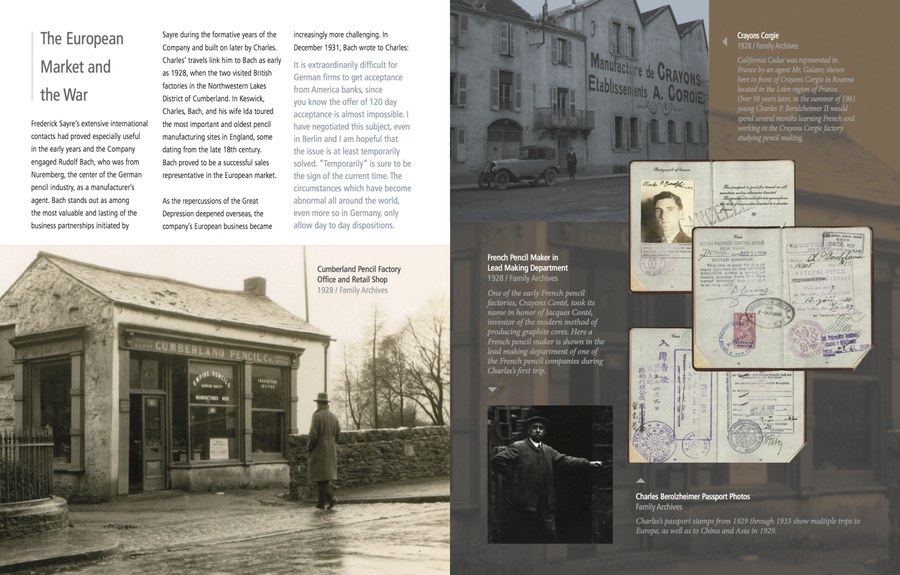The image depicts a detailed brochure or informational booklet with the main heading "The European Market and the War", chronicling various businesses that operated during the tumultuous periods of the late 1920s through the 1930s. The content details historical narratives, highlighting Frederic Says and his ventures in the French pencil and lead-making industries. On display are several vintage photographs: the Cumberland Pencil Factory, Office, and Retail Shop dated 1928, showing a man in a coat and hat walking towards the building; another image labeled "Manufacture de Crayons Establishment Corgi, 1928" featuring a crayon factory with an old car in front and another suited man in a top hat near the entrance. The photographs are complemented with historical documents such as passports and ID photos, including one of Charles Venezuela, further enriching the narrative of European businesses during the pre-World War II era.